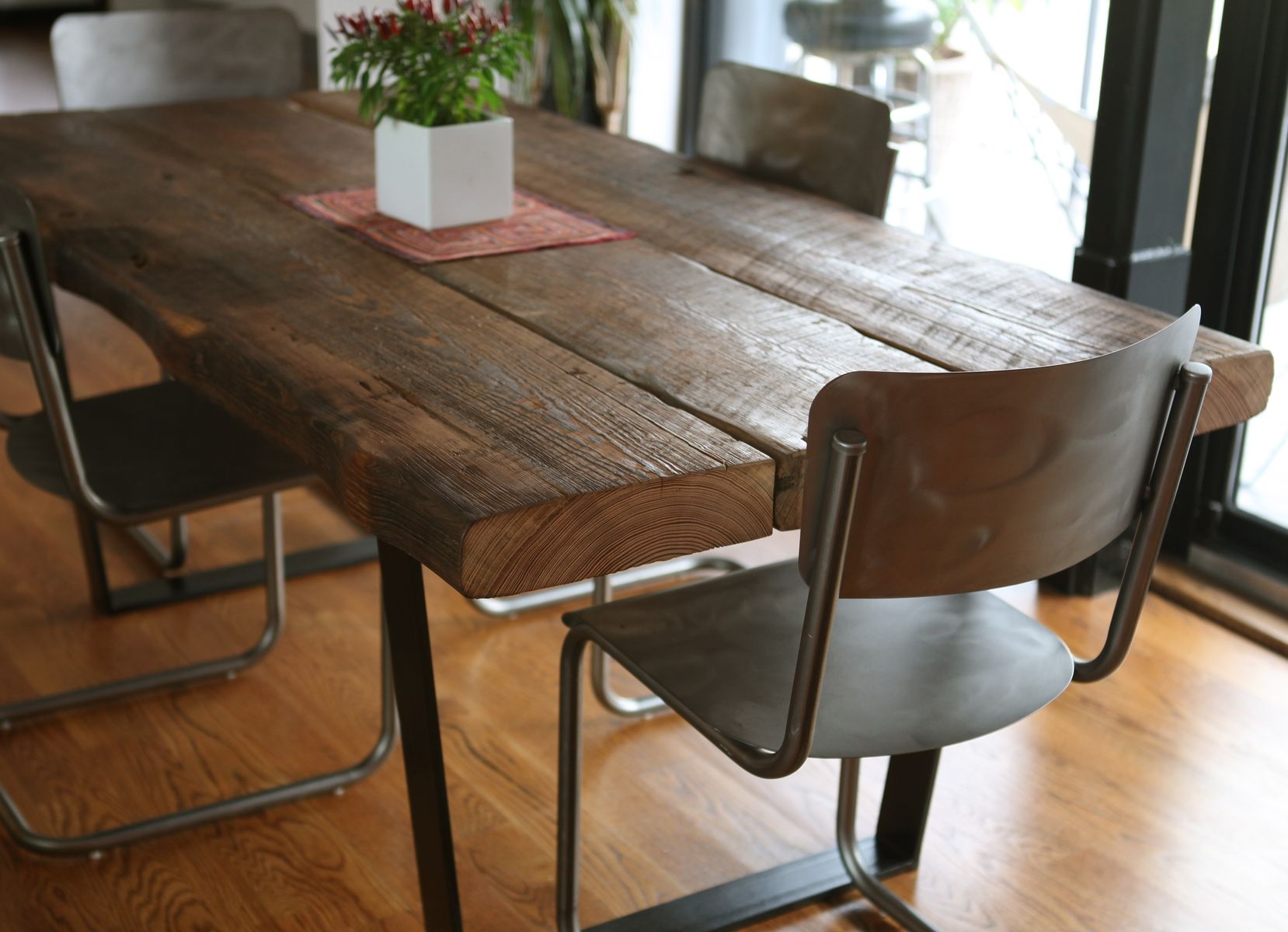This photograph captures a traditional dining room setting featuring a robust wooden table made of three thick, dark-stained planks. The table is surrounded by four metal chairs, characterized by their industrial design with wrought iron legs and bent backs, complemented by wooden slat backrests and platforms for seats. These chairs lack cushions, further reinforcing their industrial aesthetic. The table is adorned with a small square pot containing a potted plant, notable for its vibrant green leaves and delicate purple flowers, sitting on a salmon-colored mat at the center. The dining setup is positioned on a highly polished, lighter-colored wooden floor, which contrasts with the dark hue of the table. The room includes a large picture window with gray dividers, adding a modern touch to the otherwise rustic and industrial ambiance of the space.